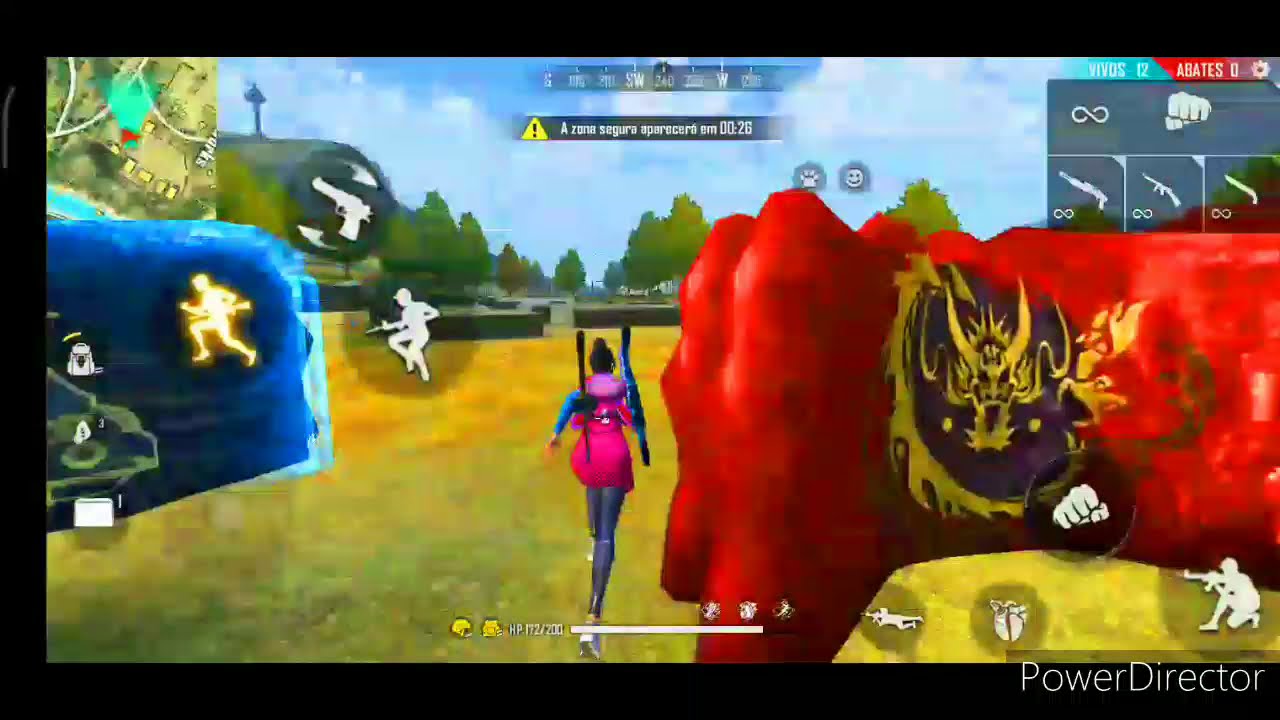The image appears to be a screenshot from a pixelated video game akin to Fortnite. Central to the image is the back of a female character wearing a pink and purplish dress with tight pants underneath and gray leggings. She has blue sleeves, white shoes, and is carrying two long rifles slung over her shoulders. As she runs away from the viewer in a yellow field marked by a hedge maze in the background, she is flanked by two large, rock-like structures: a red rock face on the right with a Viking-like symbol featuring a yellow dragon's head with horns on a purple background, and a blue rock face on the left. The scene also contains several white figures wielding guns; one is prone on his belly, facing left, while another is kneeling. The gaming interface includes a map in the upper left corner, weapon and control icons in the upper right, and a score display in the top center. The lower right corner bears the text "Power Director."